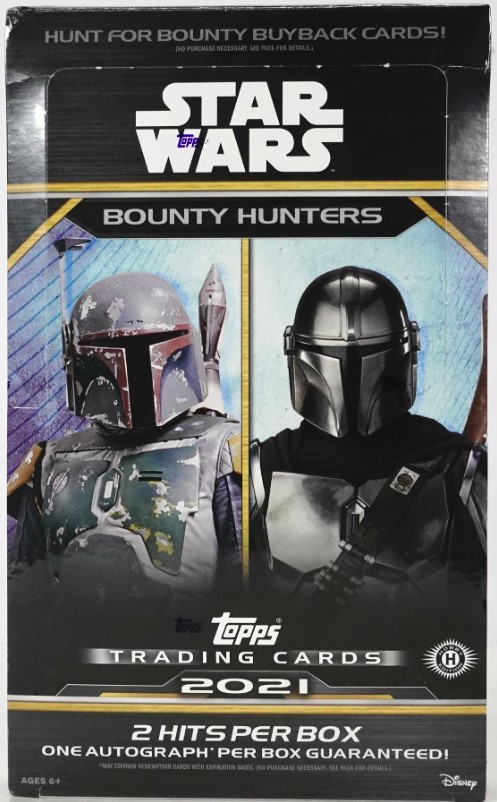The image depicts the outer packaging of Star Wars trading cards from Tops Trading Cards, 2021. The box is rectangular, reminiscent of a VHS case. At the top, the text reads "Hunt for Bounty Buy Back Cards, Star Wars Bounty Hunters," with the T.O.P.S. logo subtly integrated above the 'W' in Star Wars. Beneath, it promises "two hits per box" and "one autograph per box guaranteed," and includes the Disney logo and age recommendation "ages six plus." The central imagery features two Star Wars characters: on the left is Boba Fett in distressed white armor with a missile on his back, while on the right is an enigmatic black-armored bounty hunter with a shiny surface and a bullet casing strap across their chest.